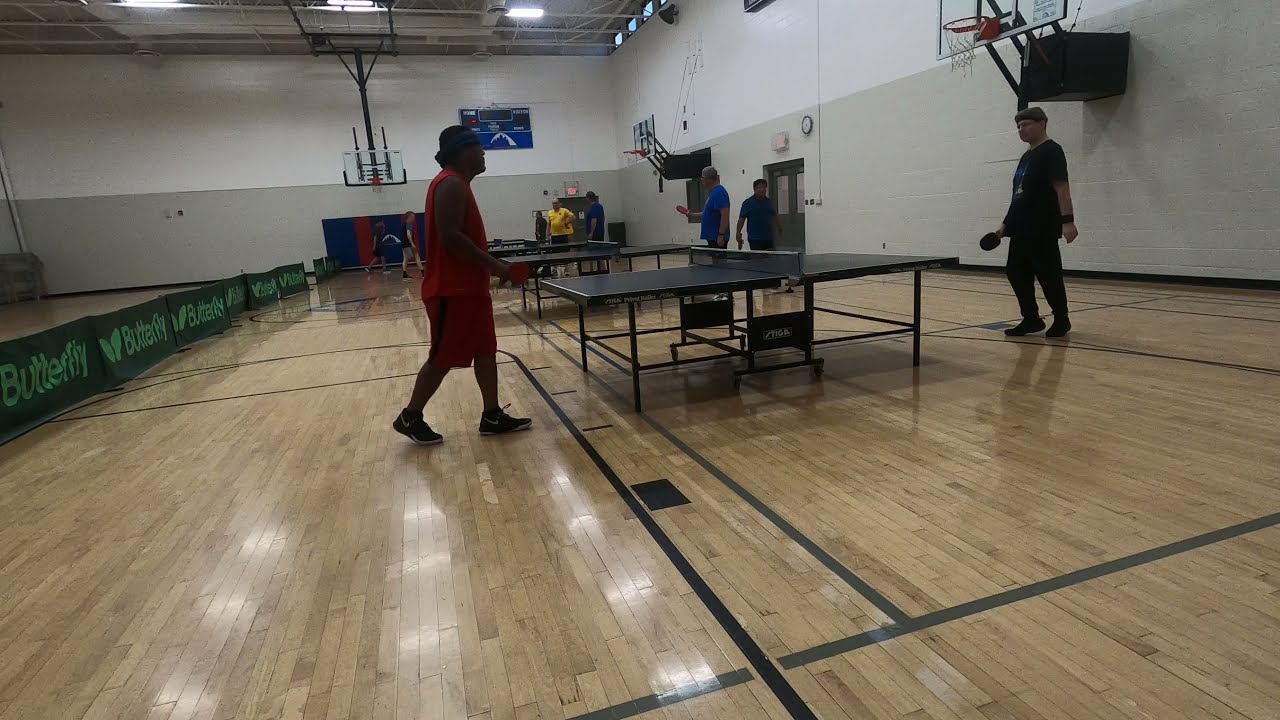The image captures a bustling scene inside a large gymnasium, where several men are engaged in spirited games of ping-pong at three tables lined back-to-back. The gym's high cement walls are painted with a light greenish-gray color on the bottom half and light gray on the top half, adorned with basketball hoops and a distant scoreboard. The light brown, glossy, rectangular wooden floor stretches toward the horizon. 

In the foreground, two men at the nearest table are playing ping-pong, one dressed in a red shirt and shorts, and the other in a blue shirt and dark pants, both holding their paddles. Behind them, additional players populate the other tables, including a man in a blue shirt on the left and another man standing in front of two doors on the right. A green mesh fence runs along the left side of the image, bordering a stage with green cloth signs that read "Butterfly." The overall scene captures the energetic atmosphere of a multi-functional gym filled with ping-pong enthusiasts.